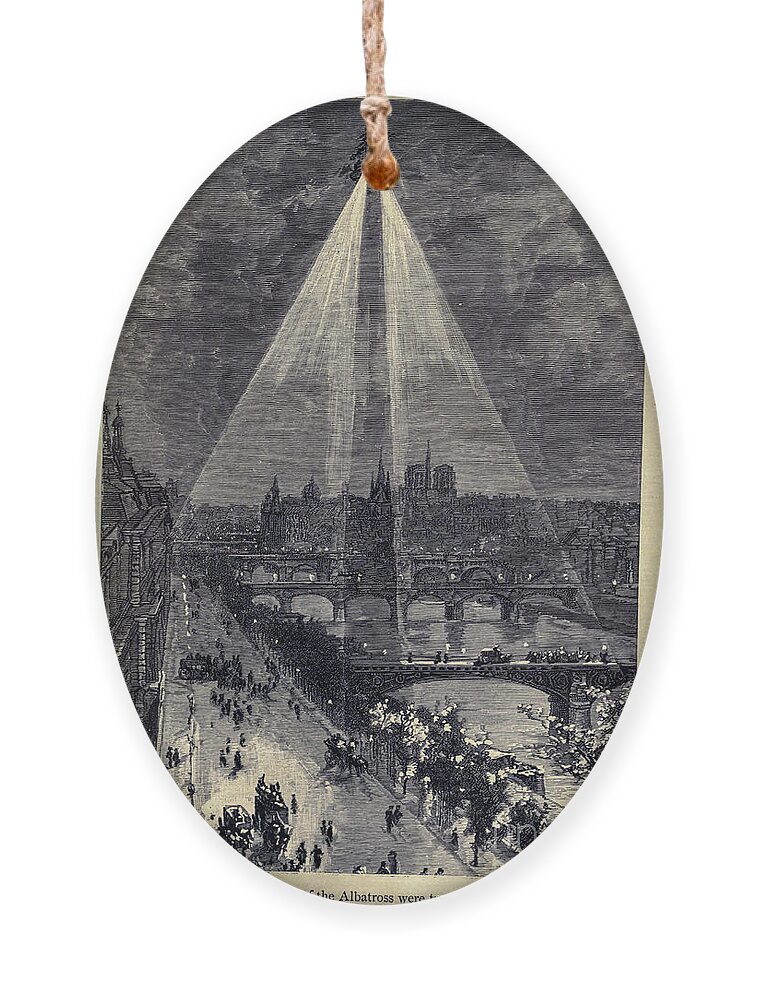The image features an intricately designed oval pendant, taller than it is wide, with no background color or border. The pendant has a predominantly gray, possibly textured stone surface, adorned with cream or ivory-colored, intricate detailing. Suspended from the top is a cream-colored, thin rope or thick threaded knot with a small, maroonish-brown bead-like circle at the end. The design on the pendant depicts a detailed cityscape with tall buildings, a river or canal with several arched bridges, and a blend of black, white, and shades of beige. The scene includes elements like old-fashioned cars, pedestrians, and people on horseback crossing the bridges, with trees lining the riverbanks. The upper half of the pendant features a plain sky where faint, triangular, conical patterns appear to shine down over the scene, reminiscent of spotlights, yet they do not obscure the intricate details below.